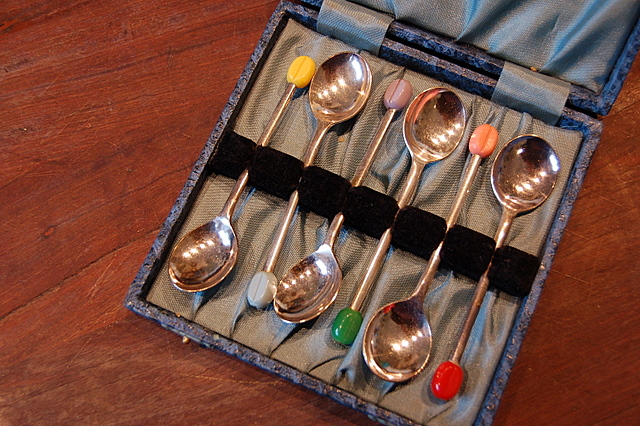This detailed photograph captures a set of six antique copper spoons displayed in a specially made, elegant case. The spoons, each with a wide, oval head, are carefully secured by individual black dividers within the box. Each spoon is distinguished by a unique, colorful plastic bead at its tip: the first spoon has a yellow bead, the second gray, the third light purple, the fourth green, the fifth orange, and the last one red. The spoons rest on a brown silky fabric lining, which complements their dark brown, coppery sheen. The outer edge of the display case is adorned with a shiny blue fabric. This refined case is placed on a rustic, worn red wooden surface, emphasizing the antique nature and careful maintenance of this exquisite spoon collection.